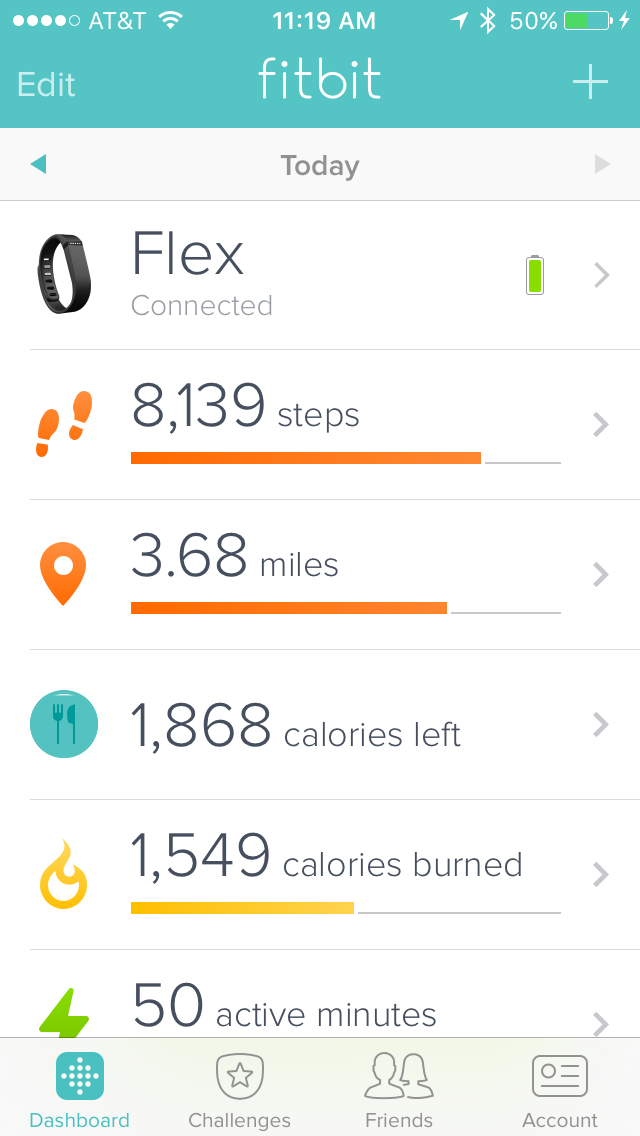This image is a detailed screenshot taken from an iPhone showcasing the Fitbit app, specifically the Fitbit Flex wearable fitness tracker. At the top, there is a light aqua blue bar with "Fitbit" on the left side along with an "Edit" button and a plus symbol on the right. Below the bar, the app displays "Today" and confirms the Fitbit Flex model is connected with full battery life. The main part of the screen displays the user's fitness statistics: 8,139 steps indicated by an orange foot icon, 3.68 miles walked represented by a location pin, 1,868 calories left shown with a fork and knife in a bluish-green circle, 1,549 calories burned indicated by a flame icon, and 50 active minutes denoted by a lightning bolt symbol. At the bottom of the screen, there are options for Dashboard, Challenges, Friends, and Account. The color scheme includes blue, white, green, gray, black, orange, and yellow. The screenshot occupies the entire image, providing a clear view of the mobile app's interface and user progress for the day.